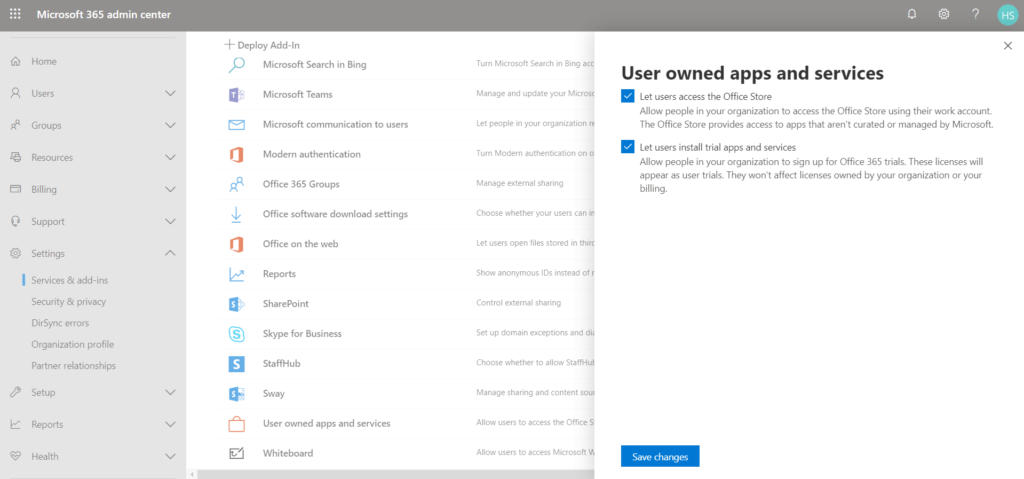The screen capture displays a section of a settings dashboard, specifically under "Reports and Health," where "Services and Add-Ins" options are showcased. On the left column, a series of expandable categories are listed. Meanwhile, the central and right portions of the screen are occupied by a list of approximately a dozen add-ins sorted in a column format.

The add-ins featured include:
1. Microsoft Search in Bing
2. Microsoft Teams
3. Microsoft Communication to Users
4. Modern Authentication
5. Office 365 Groups
6. Office Software Download Settings
7. Office on the Web Reports
8. SharePoint
9. Skype for Business
10. StaffHub
11. Sway
12. User-Owned Apps and Services
13. Whiteboard

To the right side of the screen, there is a white pop-up overlay titled "User-Owned Apps and Services." This overlay contains two checkboxes with corresponding options:
- "Let users access the Office Store"
- "Let users install trial apps and services"

Each checkbox is positioned to the left of its respective description, offering administrators precise control over user permissions related to Office services and add-ins.